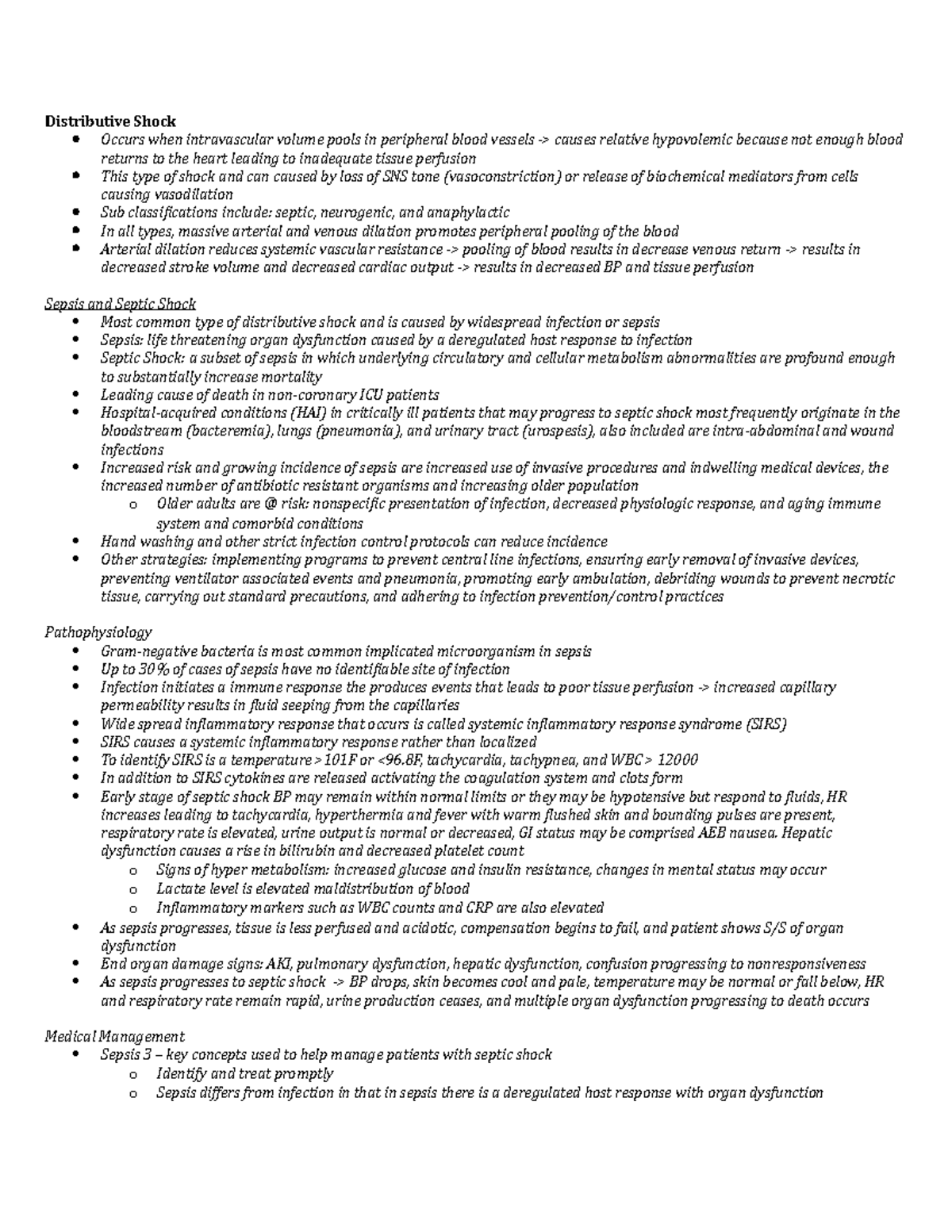Caption: 
A detailed excerpt from a medical journal webpage, presenting an extensive and technical overview of various forms of shock. The content, displayed in a meticulous bullet point format, uses solid black circles for primary bullet points and outlined circles for secondary points. The topics covered include distributive shock, sepsis, septic shock, and the medical management of sepsis. The dense, small black print packed into every line resembles an encyclopedia entry, providing in-depth medical information in a structured and systematic manner.